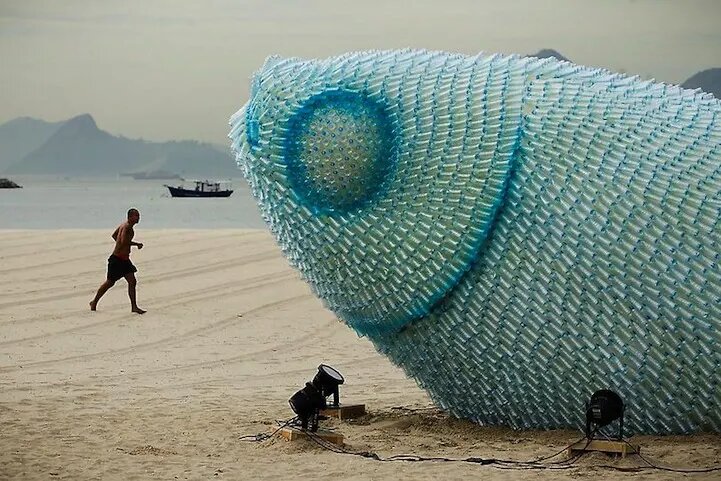This photograph captures a stunning, large-scale art installation on a beach, seemingly in South America, featuring a giant fish sculpture composed entirely of recycled plastic bottles. These bottles, predominantly bluish-green, are meticulously arranged to mimic fish scales, creating an overall teal hue that gives the sculpture a life-like quality. The fish's head, complete with a prominent upward-looking eye and visible gills, appears to be emerging from the beige sand and occupies the middle to right side of the image. Surrounding the sculpture are several footlights aimed at enhancing its visibility, although they are not illuminated in this shot.

Positioned near the impressive fish structure is a dark-skinned, shirtless man in shorts, caught mid-run with his head turned to marvel at the artistic creation. The scale of the sculpture is emphasized by the runner's presence, as the fish towers about one story high above the sandy beach. In the background, the tranquil scene extends to include open water with a few boats, and a series of hills or small mountains under a light gray-blue sky. The combination of natural and man-made elements in this image, paired with the serene yet curious atmosphere, underscores the captivating and perhaps surreal nature of this artistic and environmental statement.